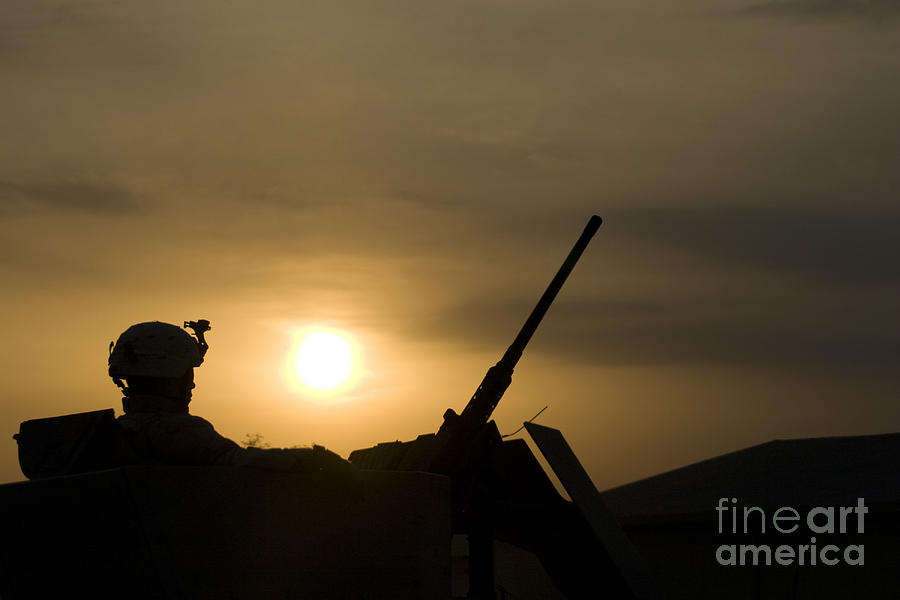The photograph captures a powerful and contemplative scene at dusk, featuring a detailed silhouette of a soldier seated in what appears to be a military vehicle, likely a tank or Jeep. The soldier, identifiable by his helmet equipped with a small camera, is framed against a backdrop of a hazy, dark orange and gray sky, with the sun setting just to the right of his head. The silhouette reveals the soldier's face, including his nose, mouth, and neck, as well as the outline of a gun nozzle pointing diagonally upward to the right. In front of the soldier, there's a faint outline of a windshield or shield. The overall image is minimalistic and dark-toned, evoking a pensive atmosphere that contrasts with its military theme. In the bottom right corner, the words "Fine Art America" are subtly inscribed in fine, white lettering, with the word "art" bolded, indicating it's an artistic piece from the mentioned group.